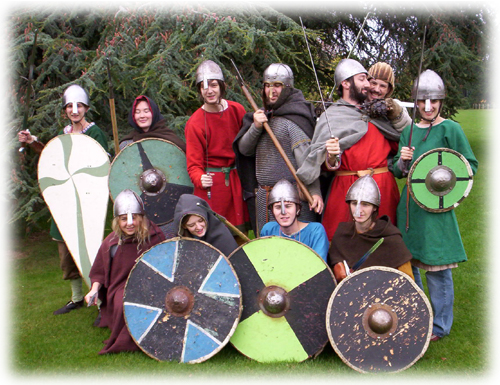The photograph captures a group of eleven people posing in medieval-style attire, each sporting silver helmets, either made of metal or foil. Arranged in two rows with seven standing in the back and four kneeling in front, all are smiling and appear to be engaging in a historical reenactment or costume event. The scene is set in a verdant park, with a green lawn beneath them and a lush backdrop of trees. Their outfits exhibit a diverse palette, including shades of grey, blue, green, black, red, and brown, adding to the medieval theme. Each individual wields various weapons like spears, sticks, a sword, and an axe, with shields prominently featuring, including one with a white and green cross. The kneeling group mirrors the medieval armament with similarly painted shields and outfits. The participants, all with light skin, evoke a sense of camaraderie and historical immersion in this picturesque outdoor setting.